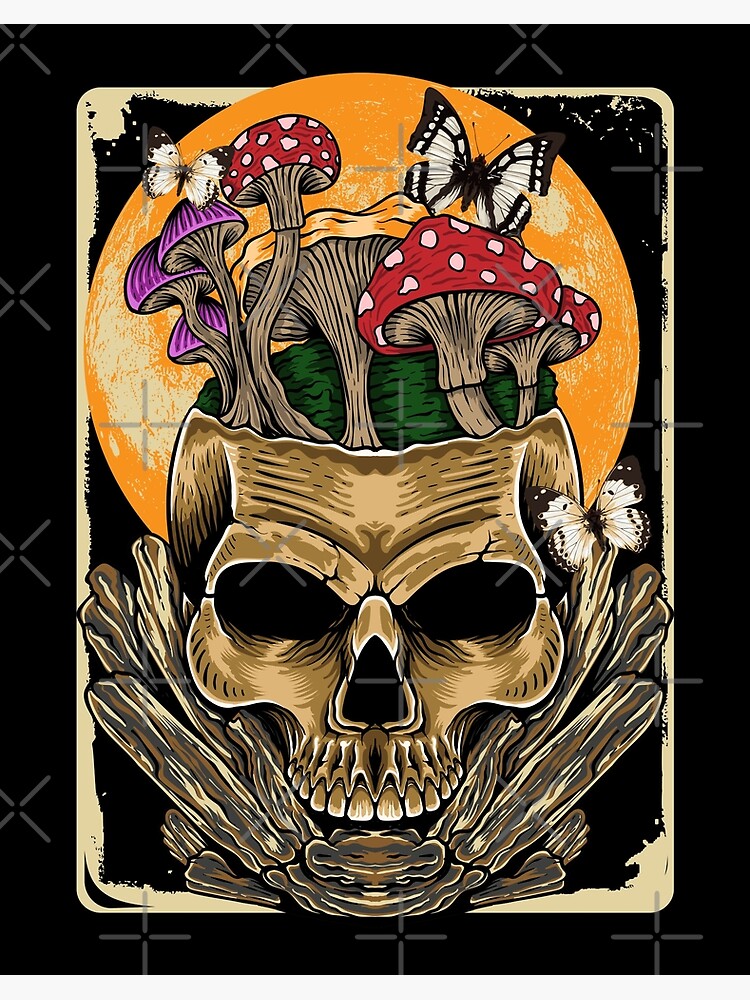This detailed artwork features a black background with a rough-edged white border framing an intriguing scene. At the center, a skull with its top removed faces the viewer, serving as the base for a variety of mushrooms emerging from the cranium. Among them, three purple mushrooms stand to the left, a red-and-white mushroom is placed in the center, followed by a large chanterelle in the middle. On the right, two more red mushrooms with white polka dots complete the array. Adorning the mushrooms and the skull are three black-and-white butterflies—two near the top and one by the right eye socket. Behind this mesmerizing display is a large, orange moon, enriching the haunting yet beautiful composition. The skull appears to be mounted on what resembles a wooden bracket, adding to the complexity of this captivating piece.